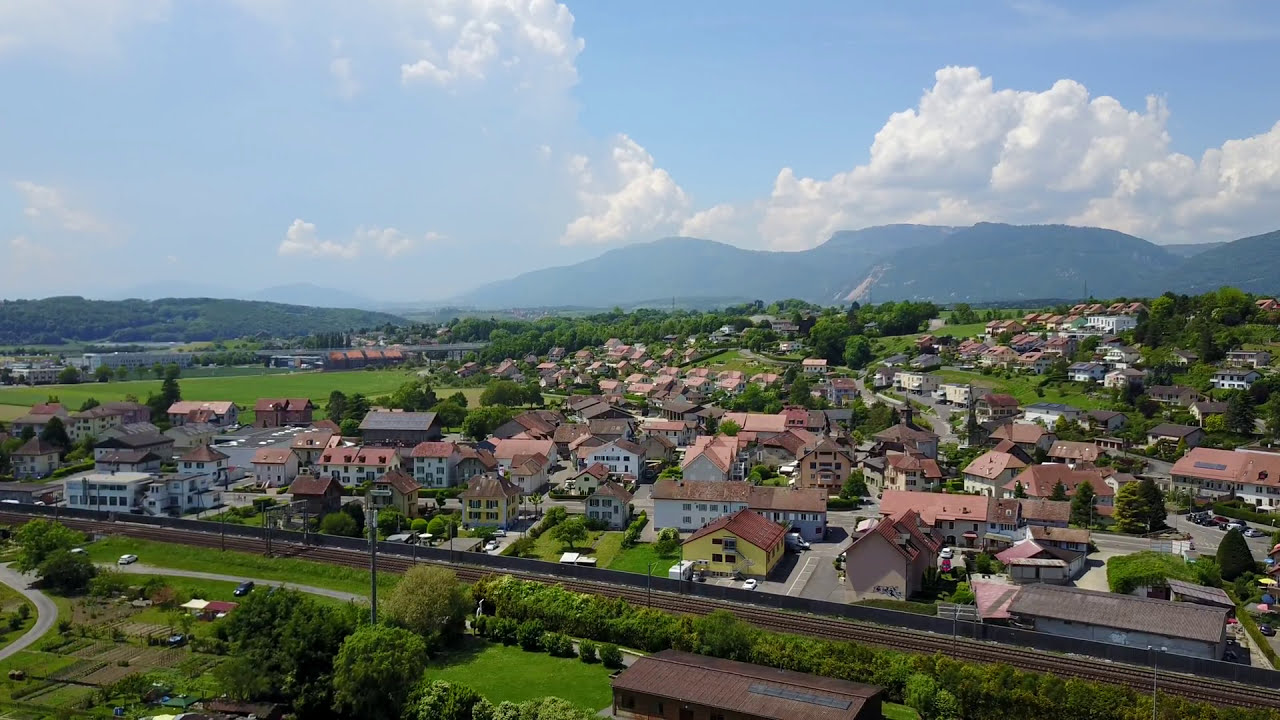This detailed aerial photograph captures a vibrant, sunlit community nestled in a picturesque landscape. The image, taken from a drone, provides a bird's-eye view of a suburban residential area characterized by numerous houses with distinctive red tile roofs. The neighborhood is surrounded by lush greenery, with well-maintained grassy fields dotting the scene. Prominent in the foreground is a railroad track, running horizontally and accompanied by additional greenery.

In the background, a magnificent mountain range with bluish-green hues rises majestically, capped by soft, white fluffy clouds against a clear blue sky. The mountain range anchors the image, giving depth to the setting. The photograph highlights the uniform yet random clustering of approximately 50 houses, signifying newer construction, and a thriving community layout. The overall scene exudes a sense of tranquility and order, emphasizing the harmonious interplay between natural elements and human habitations. The bright colors and sunny atmosphere further enhance the liveliness and clarity of the image, making it an excellent representation of residential suburban Europe.